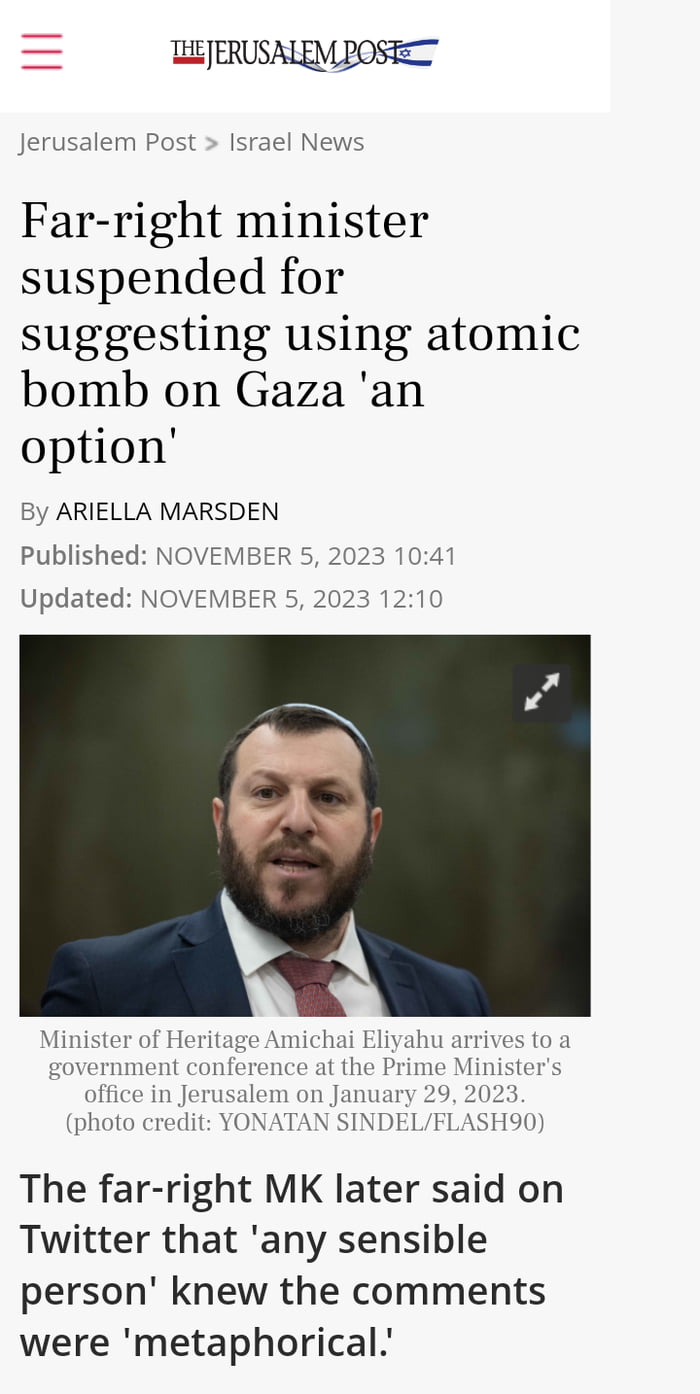The image depicts an online article layout. At the top, there is a colorful banner or header with vibrant graphics that draw attention. On the left side, there is a menu or button that suggests additional information can be accessed with a click. 

Below the header, the main title of the article is prominently displayed, followed by the names of the authors and the specific date of publication, including the day, month, and year. Scattered throughout the page are brief excerpts or snippets from the article, providing a preview of the content without revealing the full text. These excerpts are accompanied by highlight points that offer a summary of the article’s key themes and insights.

The article is presented in a standard, easy-to-read font, with black text on a white background, ensuring legibility. The overall design of the article is clean and straightforward, making it accessible and user-friendly for first-time readers.